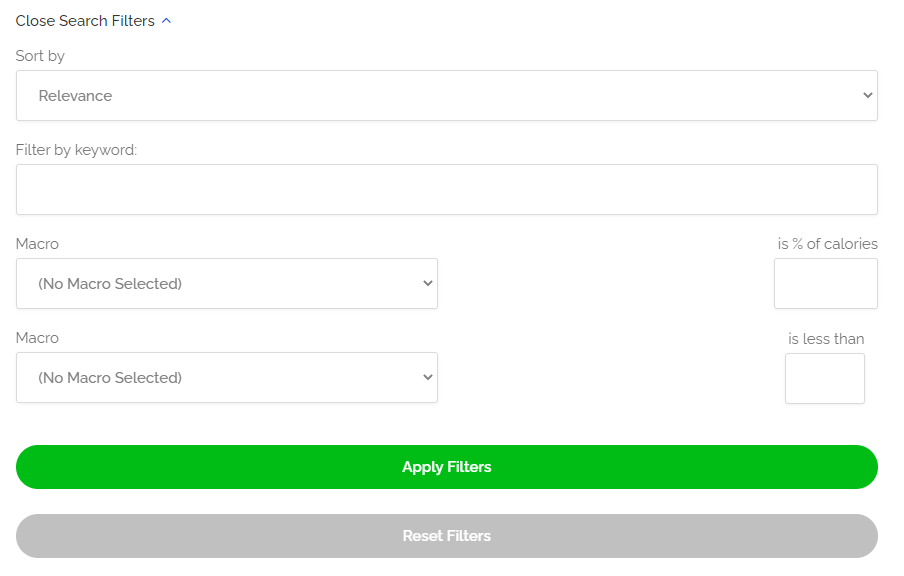The image features a minimalist interface set against a white background. Starting from the top left corner, black text reads "Close Search Filters," followed by an upward-pointing caret symbol. Below this, black text "Sort By" is displayed alongside a long white rectangular box bordered in black, with the word "Relevance" inside it. To the right of this box, there is a downward-pointing caret, indicating a dropdown menu.

Further down, the interface displays "Filter by Keyword" in black text above another white rectangular box, similar in style but empty. Below this on the left, the word "Macro" is displayed, followed by a shorter rectangular box that stretches halfway across the page, containing the text "No macro selected" along with a dropdown caret on its right edge. On the right side of this section, the text "is percentage of calories" is shown next to another empty rectangular box.

Moving down again, the left side contains the word "Macro" once more, followed by an identical rectangular box to the one above, also containing "No macro selected." Opposite this, on the right side, the text "is less than" appears next to another empty black-bordered rectangular box.

At the bottom of the page, a prominent, almost neon green tab spans the width of the page, displaying "Apply Filters" in white text. Approximately half an inch below this green tab, a gray tab of the same width is seen with "Reset Filters" also written in white.